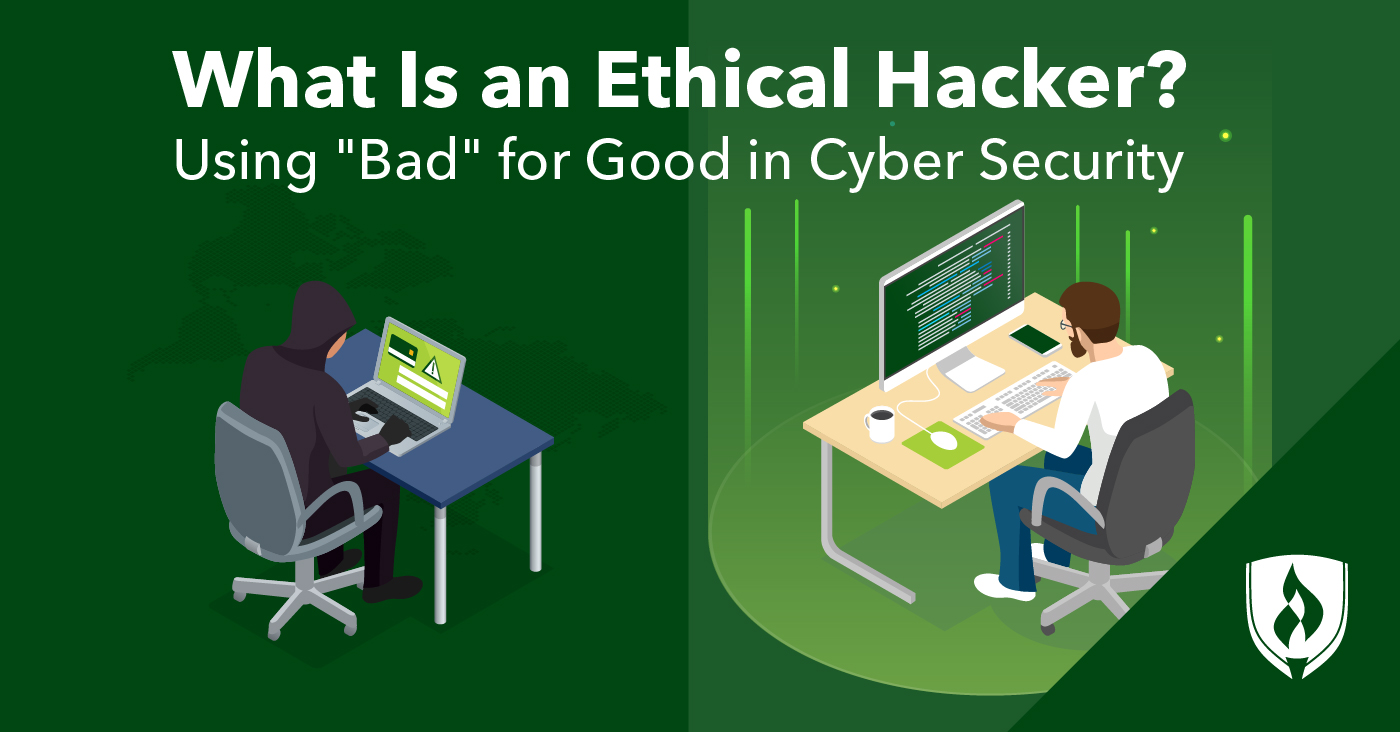This is a cartoon infographic with a green background, showcasing the concept of an ethical hacker. At the top, in bold white text, it reads "What is an Ethical Hacker?" followed by the phrase "Using 'bad' for good in cybersecurity." The infographic is divided into two halves. On the left, a dark-clad figure sits at a blue table with a laptop, displaying a triangle exclamation mark on the screen—this person, wearing a hoodie with the hood up, represents the 'bad' side. On the right, under a beam of light, is a bearded man with glasses, dressed in a white shirt and jeans, working at a larger, well-lit desktop setup with coffee and a mouse on a tan desk. A white shield emblem with a torch inside is located in the lower right corner, symbolizing protection and security. This infographic uses contrasting colors and imagery to highlight the ethical hacking concept, with the darker theme on the left and a brighter, more secure atmosphere on the right.